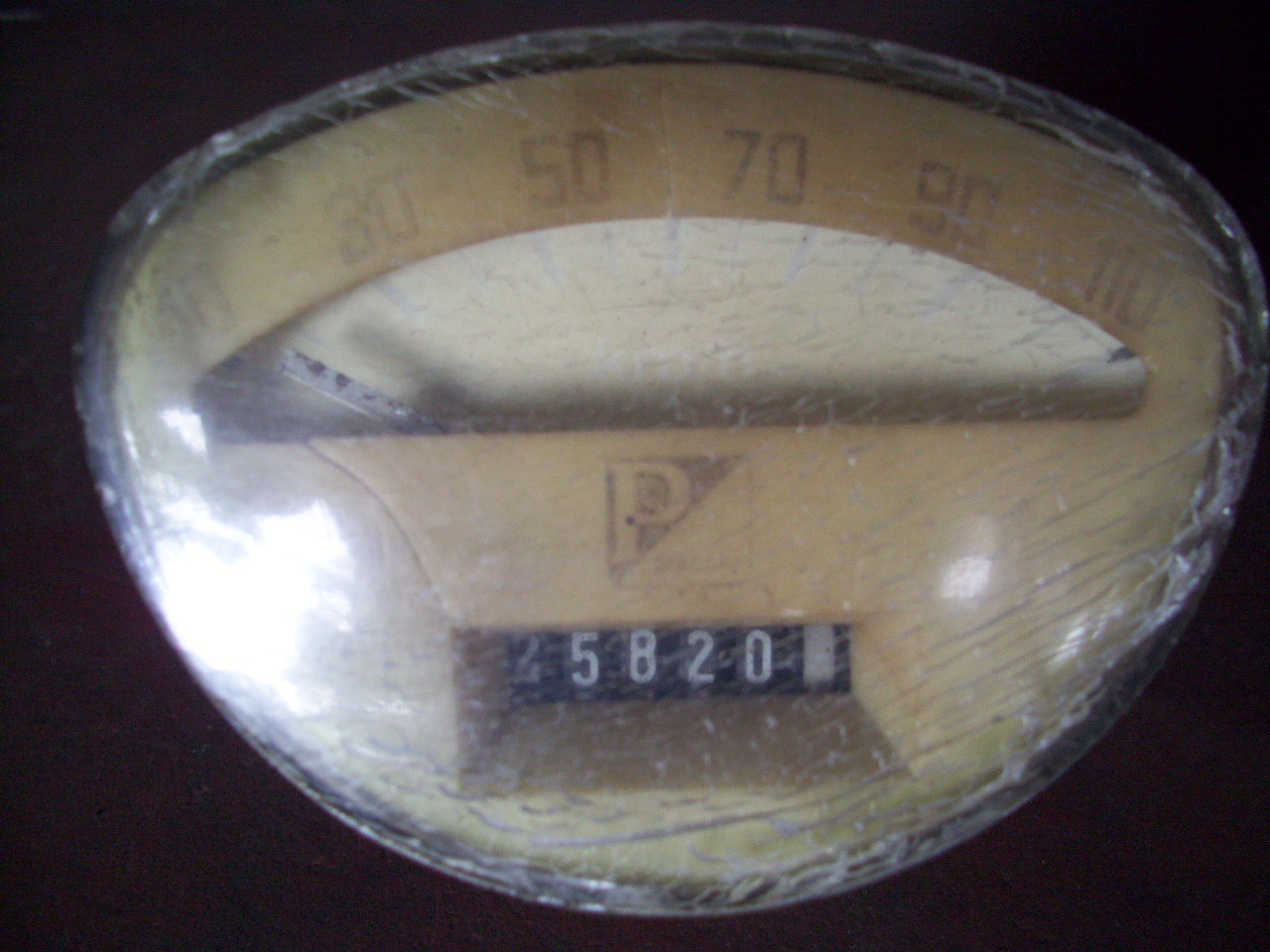The image depicts a speedometer set against a backdrop intended to be black, but appearing more as a dark red. The speedometer dominates approximately 80% of the image, taking up most of the screen. It is encased in cracked glass, evident from the multiple fissures seen on the surface. 

In the lower center of the speedometer, a "P" symbol is clearly visible, enclosed in a box with one half shaded, which seems to indicate a logo. Below this "P" symbol, in the bottom left area, the number "25,820" is displayed, likely representing the total miles the vehicle has been driven.

Above the "P" symbol, in the top center, a numbered dial ranges from 10 to 110, likely representing the vehicle's speed in miles per hour. Currently, the needle is pointing to 10, indicating the vehicle is moving at a low speed.